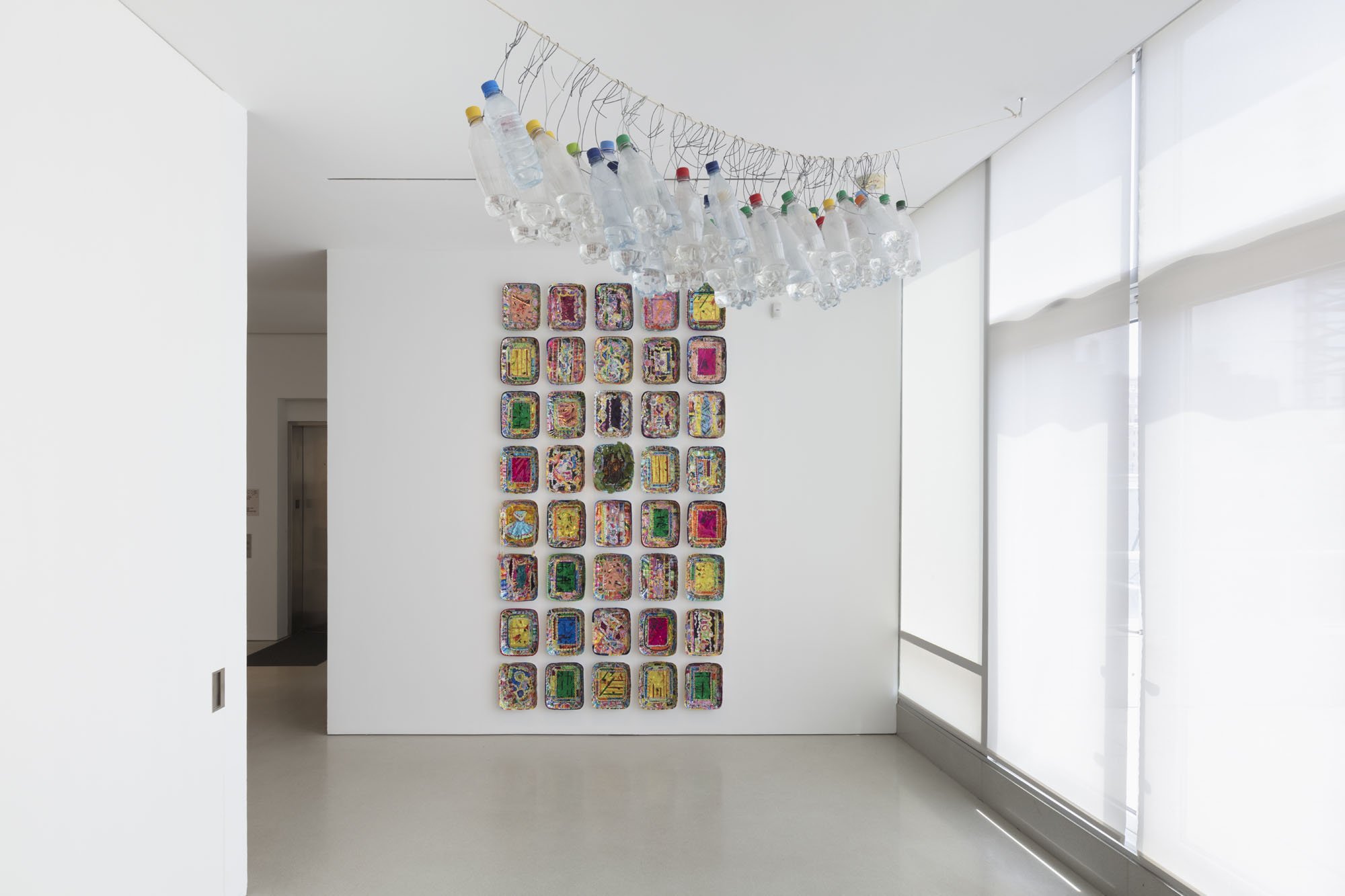This photograph depicts a section of a minimalist art gallery, marked by its clean, simple aesthetic which emphasizes the intriguing displays within. The primary focus is a white wall set against a smooth beige floor, illuminated by natural light filtering through white shades covering the right-side windows. This creates a soft, diffuse glow across the scene.

Central to the photograph is a striking arrangement of colorful trays mounted on the white wall. These trays are systematically organized into eight vertical rows, with five trays per row, totaling 40 trays. Each tray is a different vibrant color, with shades including deep magenta, turquoise, yellow, and green, resembling an array of rectangular jewels. This meticulous grid formation provides a sense of order and symmetry.

Suspended above this display is an overhead installation consisting of numerous plastic bottles, each dangling from wires attached to the ceiling. These bottles, adorned with multicolored caps - blue, yellow, green, red - add a playful, dynamic element to the otherwise serene and structured environment.

The overall scene is evocative of a contemporary museum space, designed to slow the viewer's gaze and draw attention to the colorful, peculiar objects, set starkly against the minimalist backdrop.